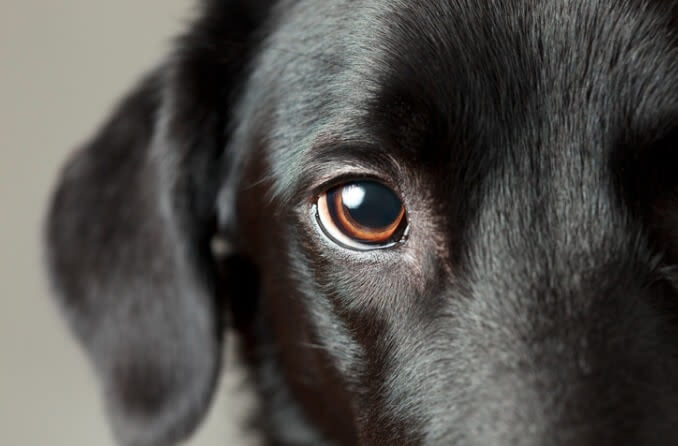This image captures a close-up of a beautiful black Labrador-type dog, with a focus on its soulful brown right eye and the right side of its head. The dog's black and shiny coat gleams, emphasizing its healthy fur. The photograph reveals the dog's right ear, part of its forehead, and a bit of its muzzle, but the left side of its face and its nose are out of the frame. The background is blurred, highlighting the sharp detail of the dog's eye, which reflects light and showcases the crisp white of its eye, lending it a youthful and vibrant appearance. Small details, such as the dog's eyelashes, add to the serene and focused expression as it gazes directly at the camera.